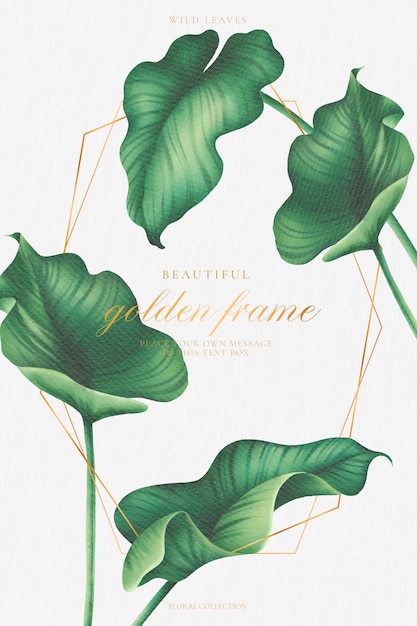The flyer we're examining features a sophisticated and delicately illustrated template titled "Wild Leaves." Set against a white background, the central design comprises four Monstera leaves sketched in varying shades of green, ranging from light to dark. These leaves are artistically arranged in different angles, forming an oval shape. They are elegantly connected and accentuated with geometrical gold details. At the very top of the flyer, in small, gold, calligraphic text, it reads "Wild Leaves." In the center, there is a prominent, beautifully presented golden calligraphic text box that states, "Beautiful golden frame," accompanied by the instruction, "Place your own message in this text box." At the very bottom, a similar text box reads, "Floral Collection." This richly colored, gold-accented flyer appears to be a template, perhaps from a website, designed for users to customize with their own information.